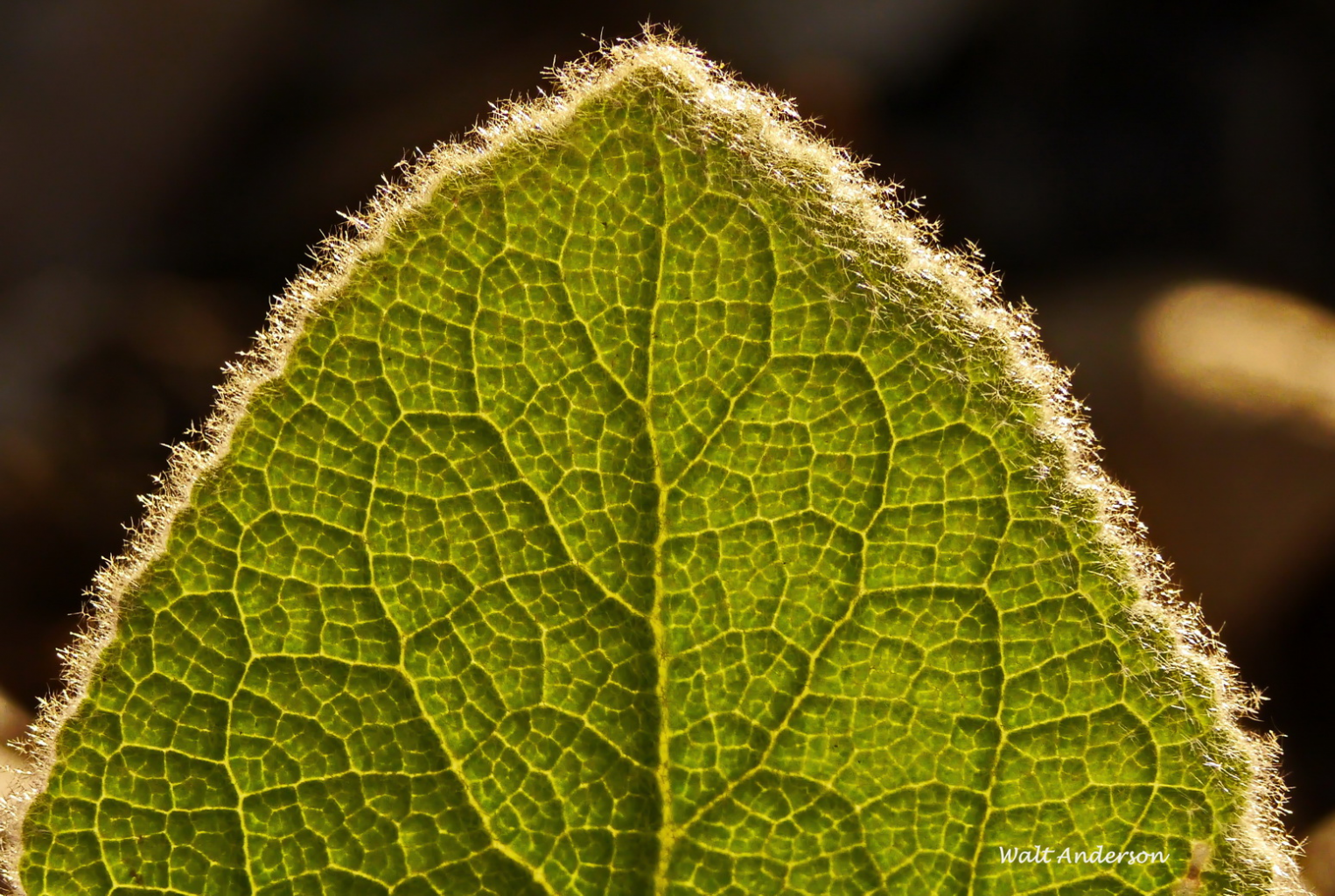This extremely close-up photograph, possibly taken under a microscope, showcases a highly detailed, triangular-shaped green leaf with intricate vein patterns. The leaf is the central focus, sharply in view, while the background is blurred and dark, with some light spots suggesting attempts of light breaking through. The veins of the leaf are prominently visible, with a network of yellow-tinged main veins and smaller offshoots, giving it deep texture and a three-dimensional appearance. The leaf's edges feature a distinctive white fuzziness, glowing under the backlight, adding to its textured and vibrant appearance. The overall scene is strikingly detailed and beautifully captured, with a watermark in the bottom right-hand corner reading "Walt Anderson."